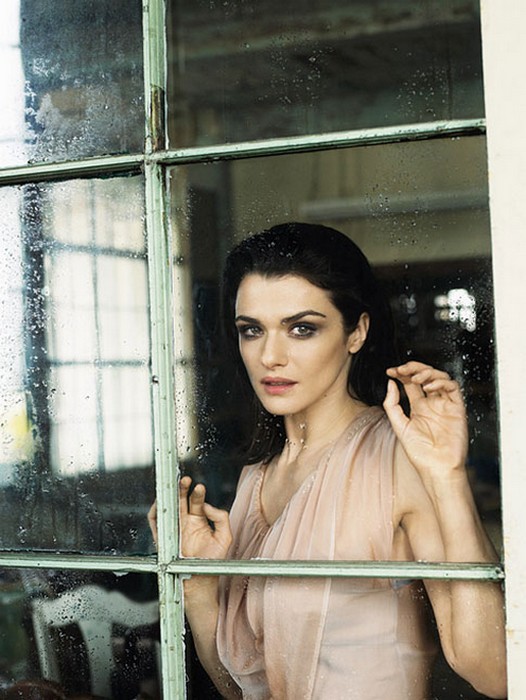In the image, a woman with long, dark brunette hair and coral-colored lips stands inside a dimly lit house, gazing out through a large, weathered window with green-painted panes. Her hair is tucked behind one ear, while her expressive brown eyes and slightly open mouth give her a look of introspective seriousness. She has on brown eyeshadow and coral lipstick, complementing her sleeveless, gauzy light pink dress that drapes elegantly around her. The old window, partially covered with water droplets and chipped paint, reveals a cluttered, unkempt room behind her, featuring another window and part of a white chair. Her hands rest gently against the glass, enhancing the sense of melancholy as she looks out into the distance. The overall scene is evocative of an actress like Winona Ryder or Rachel Weisz, capturing a moment of quiet contemplation.